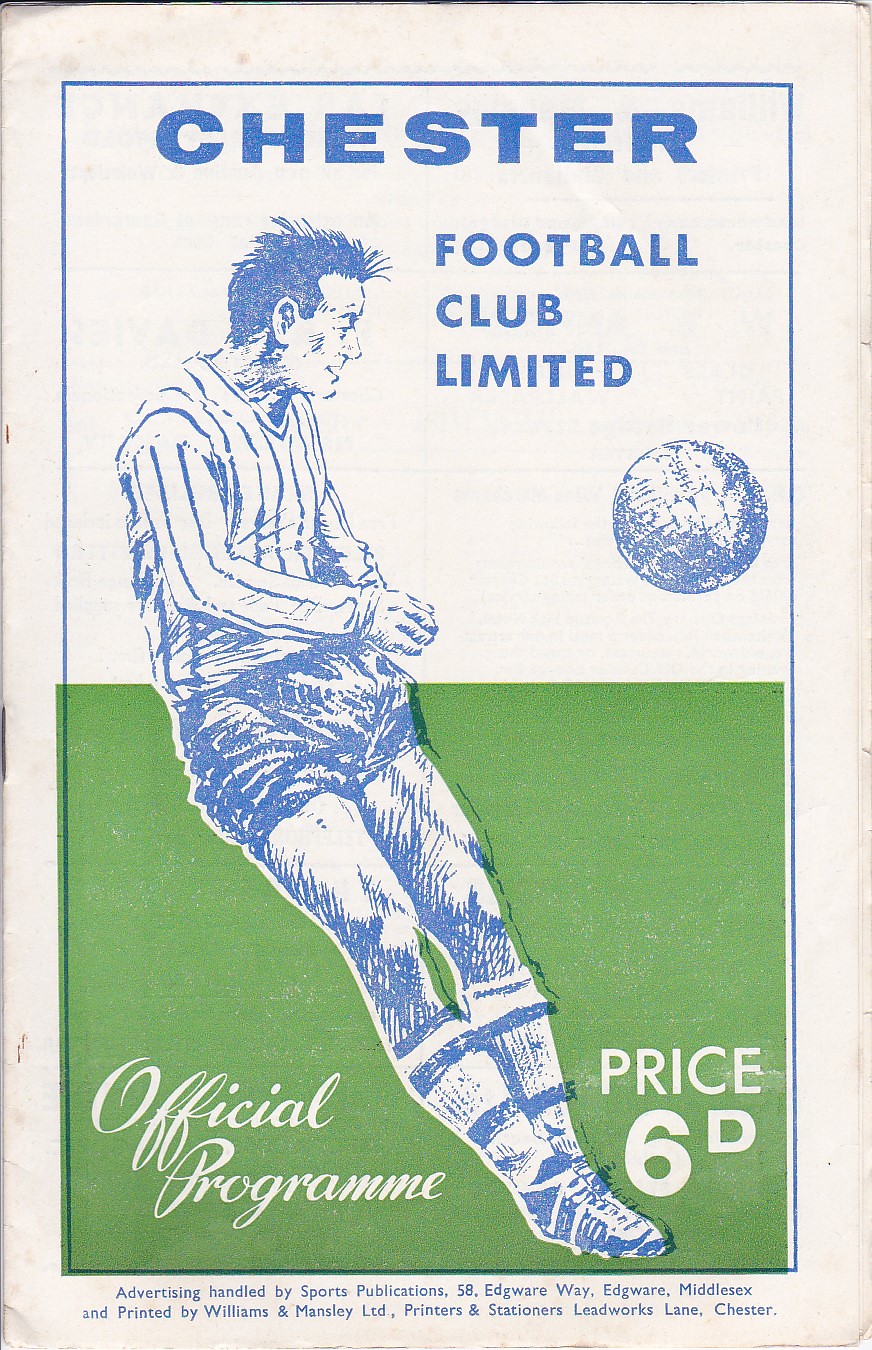This vintage-looking program cover features a soccer player rendered in a detailed pen and ink, blue and white line drawing. The player, dressed in a blue and white striped shirt, blue shorts, and blue and white striped socks, is captured mid-action with the ball suspended in midair. The background is divided into two halves, with the upper section in white and the lower section in green, symbolizing the grass field. Bold, blue text at the top prominently displays "CHESTER" with "Football Club Limited" beneath it. Additional text includes "Official Program" on the lower left and "Price 6D" on the lower right, both written in white on the green background. The program has a blue border and smaller text at the bottom detailing that it’s "Advertising Handled by Sports Publications, 58 Edgeware Way, Edgeware, Middlesex" and "Printed by Williams and Mansley LTD, Printers and Stationers, Leadworks Lane, Chester." This stapled pamphlet appears to have multiple pages, indicating it’s a comprehensive document for the event.